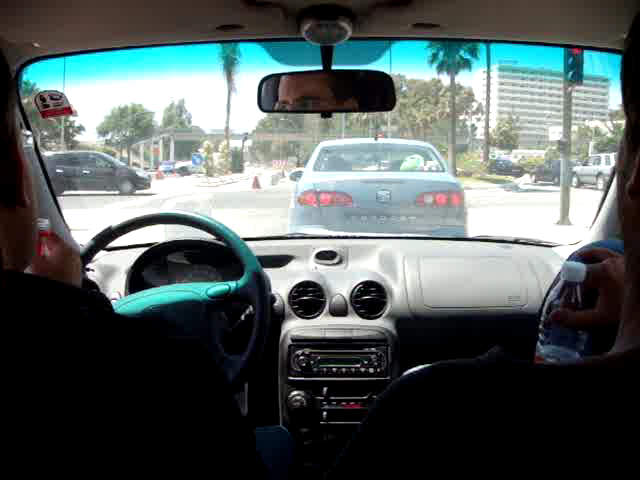This photograph captures the interior of a car from the perspective of the back seat, looking through the windshield at a city street. The image reveals two passengers in the front seats; the driver, a man with dark hair and glasses, is holding a bottle that resembles juice, and his face is partially visible in the rearview mirror. The passenger beside him has dark hair and holds a clear plastic bottle, possibly of water. The car's interior features a black dashboard and a dark turquoise steering wheel. Through the windshield, a light blue sedan is visible in front, its brake lights illuminated as it waits at a red traffic light. A minivan can be seen moving from left to right, adding to the scene of a busy intersection lined with palm trees and other types of trees, with tall buildings in the background.